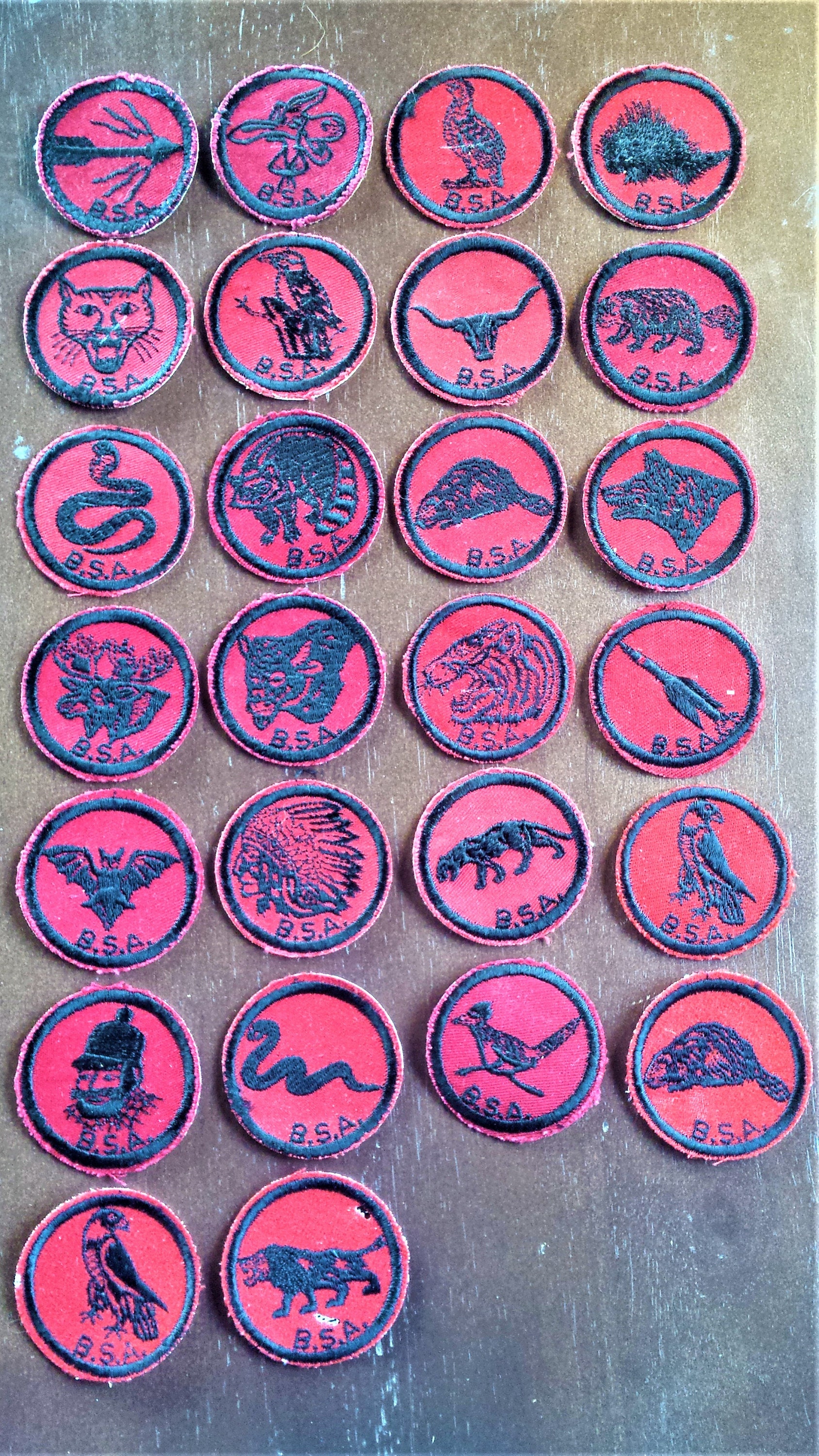This image showcases a detailed collection of circular BSA cloth badges, which appear to be sew-on patches, possibly for uniforms. The badges are arranged in four columns, with the first two columns containing seven patches each and the next two columns containing six patches each, resulting in a total of 26 patches. Each badge features a dark black symbol or depiction on a red background, encircled by a black border. The patches predominantly display various animals and symbols such as an arrow, a snake with a scale, a bird, a porcupine, a bobcat, a woodpecker, a steer, a beaver, a raccoon, a ferret, a wolf, a moose, a panther, a tiger, a dart, a bat, a Native American with a feathered headdress, a man in an outdoorsy winter hat, and a completely black snake. Underneath each symbol are the letters "BSA." The surface they are displayed on appears to be a grey, scratchy material with white specks. The patches show varying degrees of wear, with some appearing faded while others retain a brighter red, suggesting they are quite old and possibly handmade.